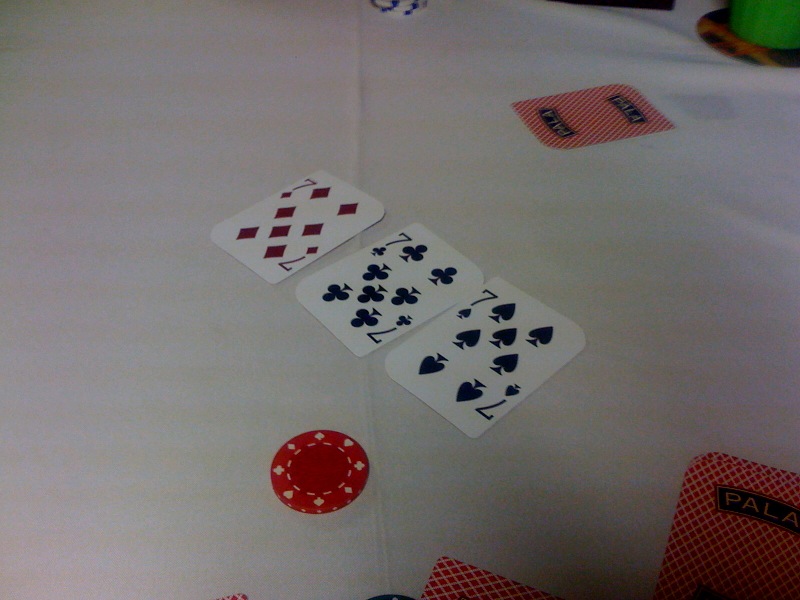A neatly set table draped with a pristine white tablecloth serves as the backdrop for a curious display of playing cards and an assortment of items. Prominently arranged on the table are three face-up cards: the seven of diamonds, the seven of clubs, and the seven of spades, aligned from left to right. Additional cards, showing only their patterned red and white backs, are scattered around the central trio. One card lies directly across from our viewpoint, while at least two others partially enter the frame from the bottom edge. The distinctive backs feature the word "Pala" in capital letters, overlaid on a design of red crisscrossing white lines. A red poker chip is aligned with the seven of spades, positioned to the far right. Intriguingly, in the upper left corner, a brown wooden coaster is visible, holding what appears to be a lime green can, likely containing a beverage, although the specific details remain obscured. The overall composition hints at a paused moment in a casual card game.